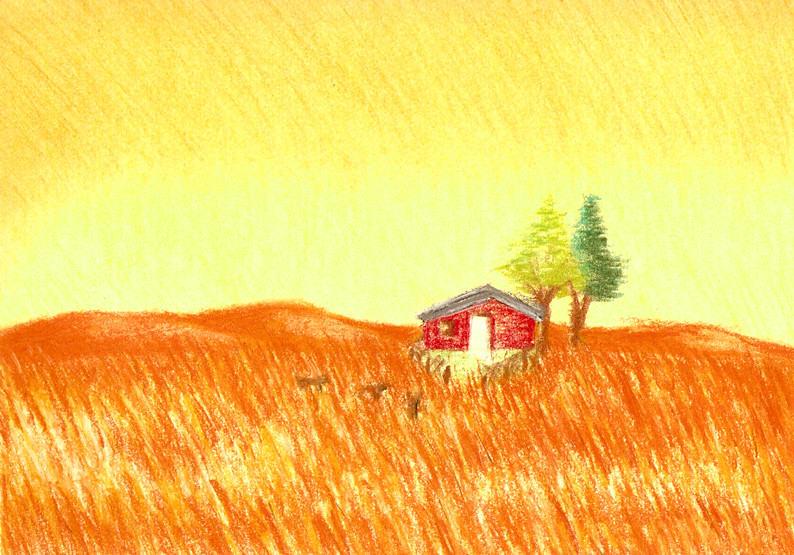This is an oil pastel drawing, likely created by a child or young adolescent, featuring a vibrant landscape composed of a range of warm and vivid colors. The sky dominates the top half of the picture, rendered in a blend of yellows that gradually shift to dark yellow at the edges, creating a vignette effect. The crayon strokes are clearly visible, giving the sky a textured, blooming appearance. The lower half of the image is a depiction of a field, colored in varying shades of oranges and yellows that suggest a field or crop growing in a paddock.

At the center of the drawing stands a small red barn with an open, white door and a grey, almost silver, roof. Adjacent to the barn is a small fence and a distinctive V-shaped pattern in front. Beside the barn are two trees: one in a lighter green, the other in a darker green, both with brown trunks. The overall composition of the pastel work uses these vivid and contrasting colors to bring to life a serene, rustic scene.